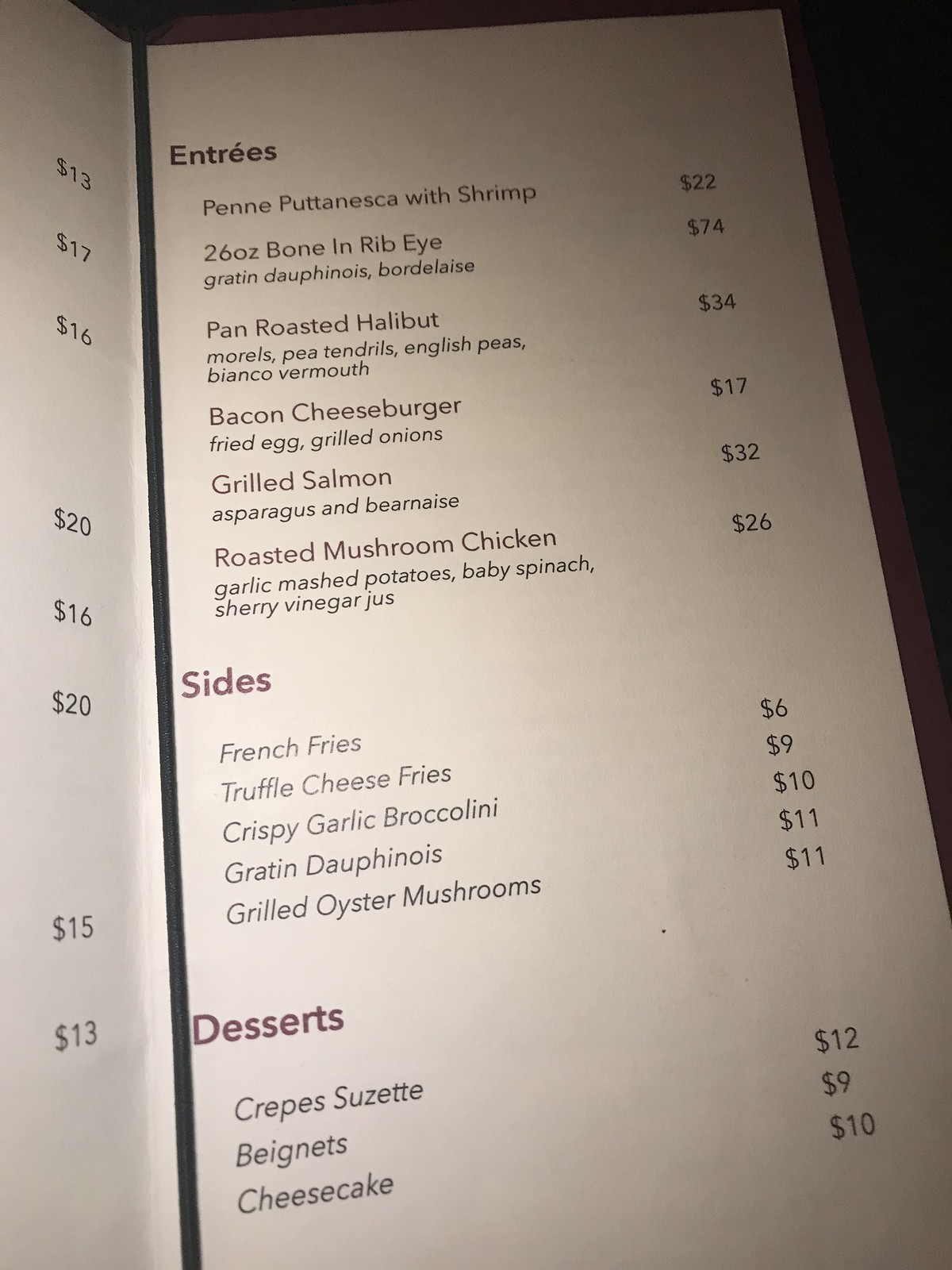In this elegantly lit image of a restaurant menu, one can discern the upscale ambiance of the establishment, likely characterized by its low lighting conducive to a refined dining experience. The menu itself is illuminated, presenting a clear view of its details despite the dim environment. 

The visible portion of the menu is bifurcated by a bold black line. On the left-hand side, one can only make out the prices, which include $13, $17, $16, $20, $16, $20, $15, and $13, though the corresponding items are not visible, hinting at a varied pricing structure possibly for appetizers or beverages. 

On the right-hand side, the menu is divided into distinct sections: entrees, sides, and desserts, with each category title highlighted in bold red font, making them stand out from the rest of the text which is in a smaller black font. The entrees listed include:

- Penne Puttanesca with Shrimp: $22
- 26 oz Bone-In Ribeye: $74
- Pan-Roasted Halibut: $34
- Bacon Cheeseburger: $17
- Grilled Salmon: $32
- Roasted Mushroom Chicken: $26

The sides, each ranging from $6 to $11, feature:

- French Fries
- Truffle Cheese Fries
- Crispy Garlic Broccolini
- Gratin de Fenouil
- Grilled Oyster Mushrooms

For desserts, the following options are listed:

- Crepes Suzette: $12
- Beignets: $9
- Cheesecake: $10

The careful wording and sophisticated layout imply that this is a menu from a high-end restaurant. Each item and price is clearly delineated, ensuring ease of selection for patrons.